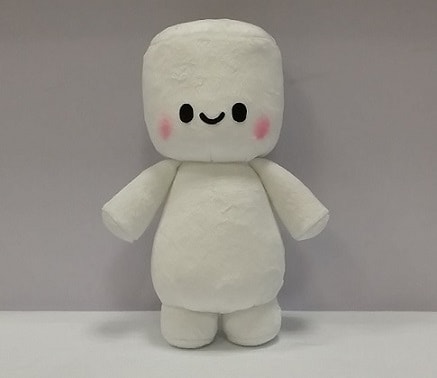A small plush doll resembling a marshmallow is positioned upright on a white table with a dark gray background. The doll has a white, square-shaped head that mimics the texture of a marshmallow. It features two small black eyes and a simple black smile, with rosy pink cheeks adding a touch of color. Its body, resembling the shape of the Diagnostic robot from Big Hero 6, is white and has a slightly inflated appearance, covered in what seems to be cotton fabric. The body narrows towards the neck, then broadens out like an hourglass, giving it a larger stomach. The doll has small, cone-shaped arms and tiny stubby legs without detailed fingers or toes. Overall, the happy expression on its face, with rosy cheeks and simple features, exudes a cheerful, cartoon-like charm, reminiscent of characters like Stay Puft the Marshmallow Man from Ghostbusters. The image focuses solely on this whimsical, child-like toy, with no other objects or text present.